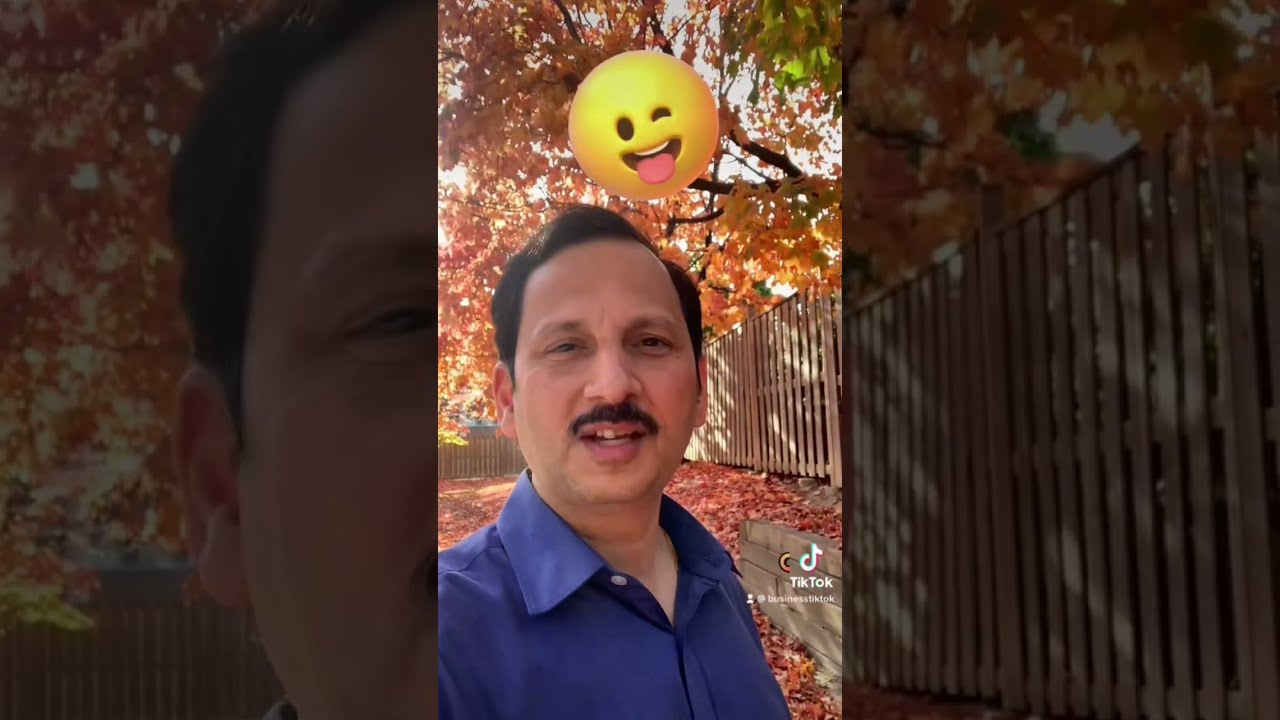In this TikTok image, a man with short black hair and a black mustache gazes forward, his body turned slightly to the right while his head tilts back to the left. He has brown skin, one eye squinting and the other open, with his mouth slightly ajar, faintly revealing his teeth. He wears a blue button-up shirt with the collar open at the top. Above his head is a white circle emoticon with its tongue sticking out, showing a hint of teeth. The background features trees adorned with orange leaves, some scattered on the ground and others still clinging to the branches. A wooden plank fence extends on the right side of the image. The scene is set in a residential area with a hazy sky overhead.

The image is presented vertically, with faded and zoomed-in sections flanking the main picture. On the far left, there's a close-up of the man's left ear, while the far right features a zoomed-in part of the wall. The top right corner of the image shows a few green leaves. At the bottom right, the TikTok logo appears, accompanied by the user’s TikTok handle. The overall aesthetic creates a collage-like effect, emphasizing the man and his surroundings.